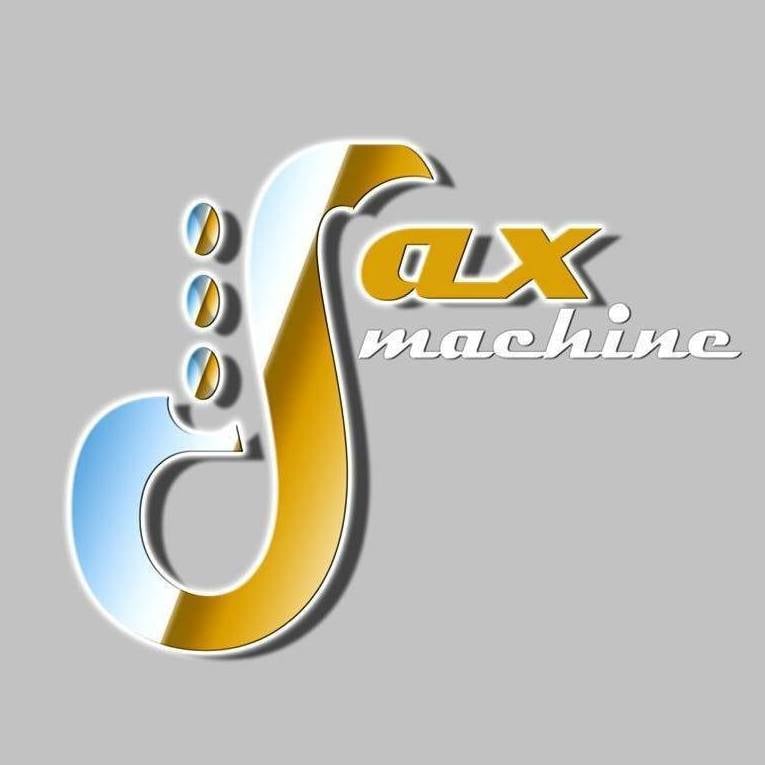This image appears to be a computer-generated brand advertisement or logo with a very minimalist yet striking design. The background is a plain shade of gray, redirecting all attention to the central logo and text. Dominating the left side of the image is an "S" designed to resemble a saxophone, complete with three vertically aligned buttons. This saxophone-inspired "S" showcases a tri-color scheme: the top portion is white, the middle segment is blue, and the lower part is gold, creating a vibrant and dynamic visual effect. The design gives the letters a 3D appearance with white outlines and black shadows. Following the "S," the letters "A" and "X" appear in gold, each outlined in white, forming the word "SAX." Below this artistic representation, the word "MACHINE" is in white lettering, invoking imagery reminiscent of fonts used by classic brands like Fender guitars. Overall, the image conveys a sleek, professional feel, suggesting that the "Sax Machine" might be a product or brand logo suitable for use on business cards or websites.